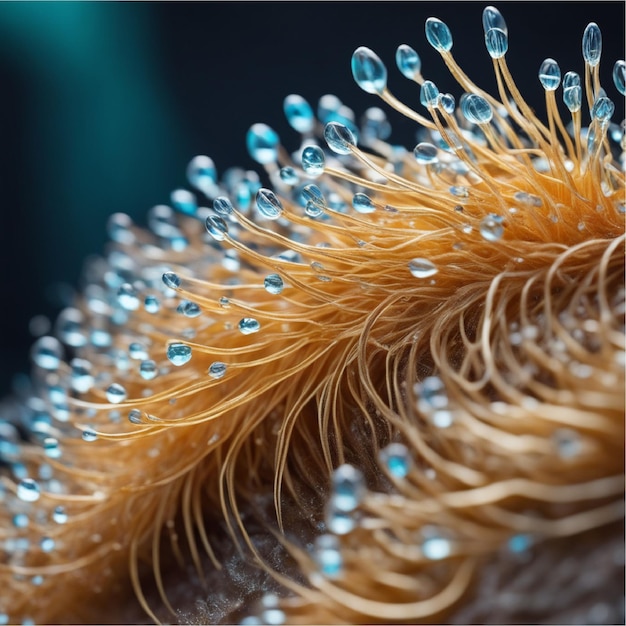The digital image features a close-up of an unknown, orangeish-yellow object that resembles skin or fur. The object has numerous stick-like, hair or fur strands with an orangish-brown gradient transitioning to light brown or yellow at the top. Each strand is adorned with a semi-translucent, blue water droplet at its end. The background is predominantly dark blue, blurred to emphasize the main subject, with a distinct light blue stripe on the left side, suggesting sunlight penetrating through a sea-like environment. The focus and microscopic view create an impression of tiny water droplets suspended delicately on the strands, adding a surreal and intricate texture to the scene.